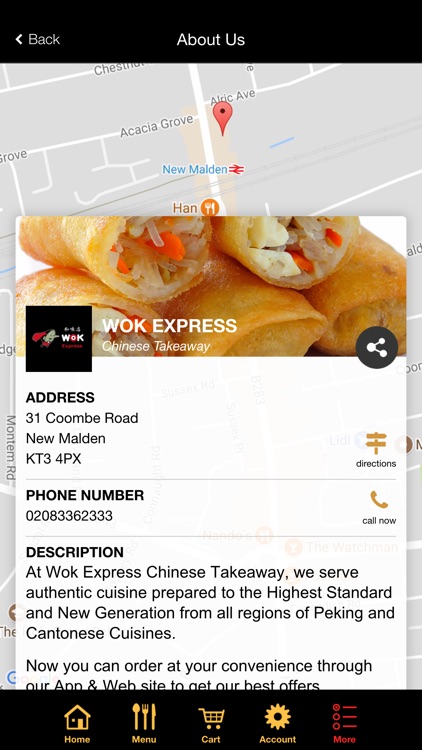Screenshot of the "About Us" section for Walk Express Chinese Takeaway:

The background features a detailed map. Prominently overlaid on the map is the Walk Express Chinese Takeaway logo. Below the logo is the address: 31 Coombe Road, New Malden, XT3 4PX (which appears to be a Canadian postal code). To the right of the address, there is a "Directions" link.

Underneath, contact information includes the phone number: 0208-336-2333, with a "Call Now" prompt adjacent to it.

The description reads: "At Walk Express Chinese Takeaway, we serve authentic cuisine prepared to the highest standard and new generation from all regions of Peking and Cantonese cuisines. Now you can order at your convenience through our app and website to get our best offers."

Beneath this text are navigational buttons labeled: Home, Menu, Cart, Account, with an additional "More" button in the bottom right corner.

At the top right corner next to the Walk Express Chinese Takeaway name, there is a "Share" button.